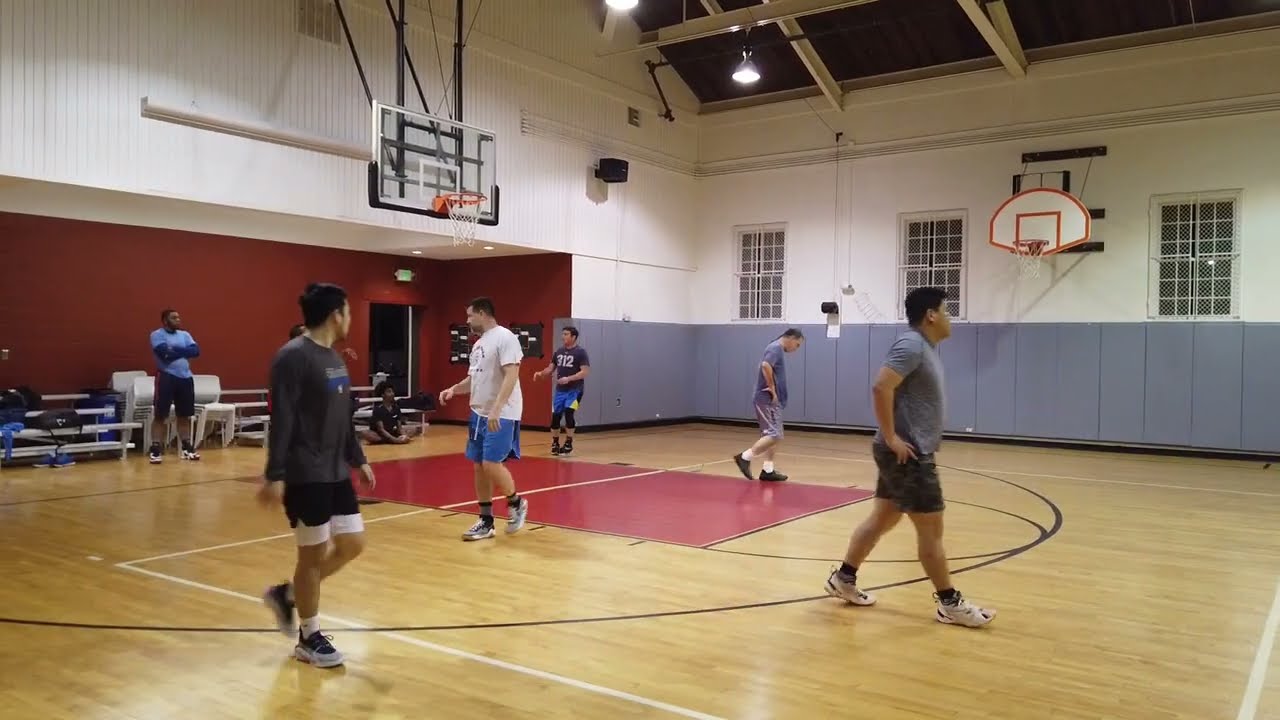The image captures a scene in a gymnasium, suggesting an informal basketball meet, possibly a practice session or a friendly game among a group of men. The wooden gym floor shines under the fluorescent lights, and we see various court markings, including a distinctive red square at the center. There are five men on the court, all in shorts and t-shirts, with some appearing as blurs in motion, indicating dynamic movement. Two men are sitting on the sideline; one cross-legged on the floor, and another in a blue shirt standing to the far left, observing the activity. In the background, the gym's architecture includes both left and right walls featuring basketball hoops with their respective backboards. The left wall showcases a white-paneled wooden surface, while the right wall presents a white and orange hoop and backboard. Windows with black and white square patterns also line the gym, hinting it might be nighttime outside despite the bright indoor lighting. One man, dressed in a grey shirt, shorts, and white trainers, walks towards the right-hand side, followed by another man moving backward. A third individual, with arms crossed, is scrutinizing the players attentively from the side, completing the lively yet casual atmosphere of this basketball setting.